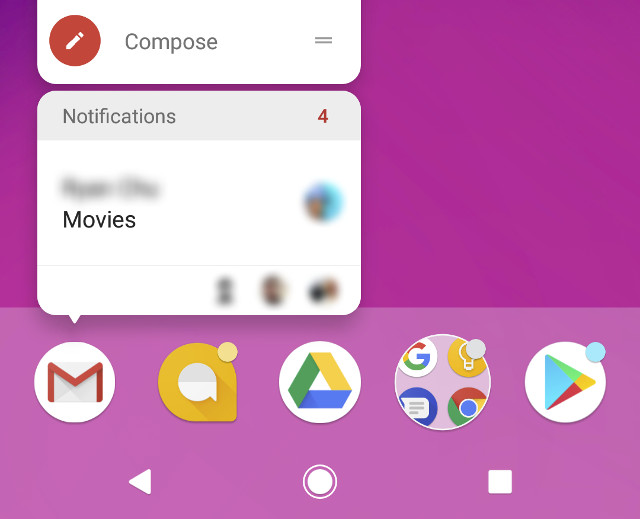This image is a detailed screenshot of the bottom part of a home page on an Android device. Starting from the bottom navigation bar, positioned in the bottom left corner is the back arrow icon. In the center, the circular home button is visible, and in the bottom right corner, there is a square icon, likely for displaying currently open windows on the device.

Above this navigation bar, there are five distinct application icons lined up. Beginning on the far left, the Gmail icon is displayed with two notification bubbles: one indicating four unread messages and another labeled "Compose". It seems the email preview shows "Movies," although the email address and sender’s name are obscured. 

Next to Gmail is a messaging app, marked with a yellow button that hints at pending notifications. Centrally placed is the Google Drive app, followed by a partially obscured icon that looks like the primary Google app. There's also an icon featuring a light bulb, the Google Chrome browser icon, and another unspecified messaging app. It is unclear if this could lead to another screen or more applications. A small gray button in one of the corners suggests either pending notifications or a potential update.

Finally, at the far right is the Google Play Store app, distinguished by a blue dot next to it, which might indicate new updates or notifications.